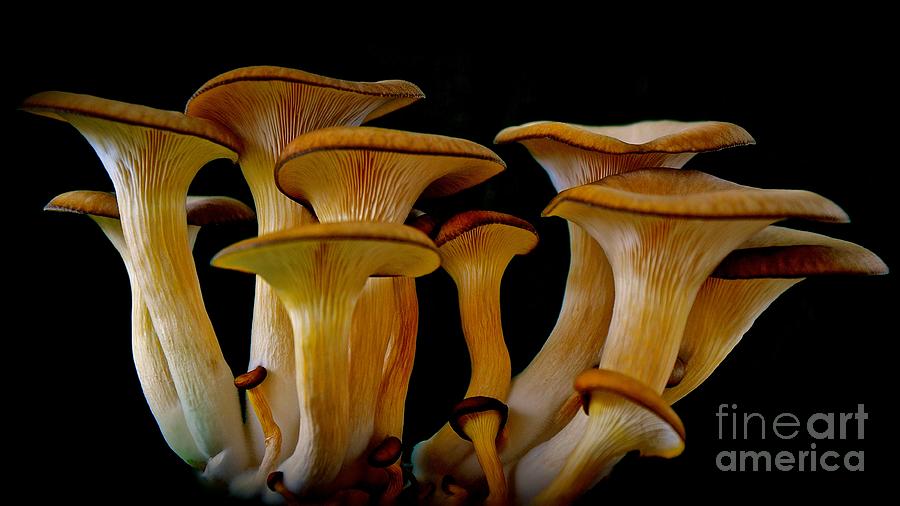The close-up image features a striking cluster of wild mushrooms, characterized by their king oyster-like appearance, which are notably consumed in Asian cultures. They appear to be growing from a single area, forming two distinct groups connected at the base. The mushrooms' wide caps are predominantly brown with a subtle red rim, and the texture is marked by bumpy, vein-like stripes. The stalks are thick and robust, supporting both large and smaller mushrooms within the groups. The background is entirely black, emphasizing the detailed and natural beauty of the fungi. The photograph, potentially captured by Fine Art America, bears their logo in the bottom right corner, indicating a professional and artistic presentation of these mushrooms.